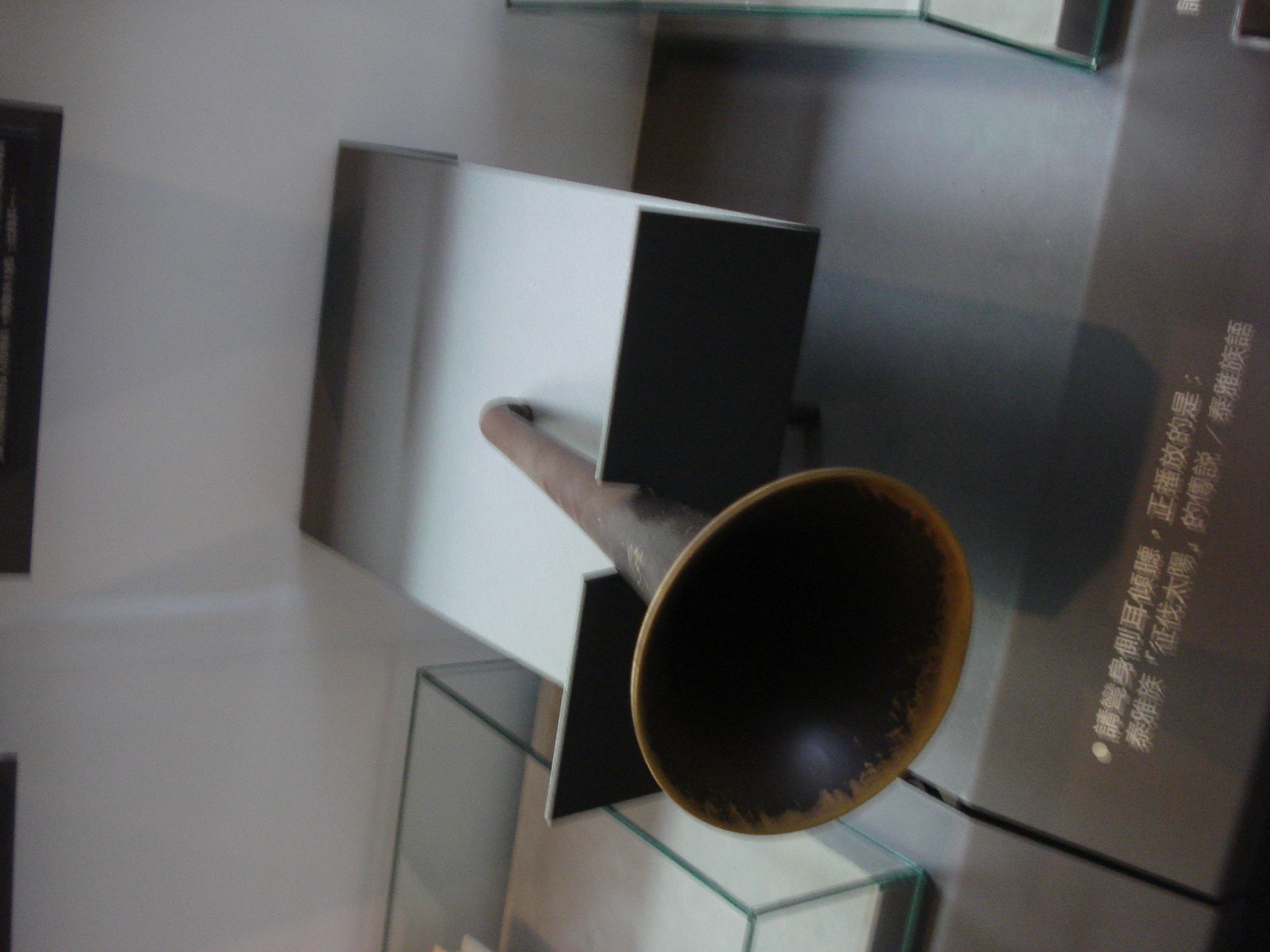This is a color photograph taken indoors and displayed in landscape orientation. The image features a museum exhibit showcasing a brass or bronze horn, supported horizontally in a notched black cardboard holder. The scene appears slightly tilted, making the horn appear to be on its side. Behind the horn is a white wall, serving as a neutral backdrop that enhances the focus on the display. The horn rests on a metal shelf that extends from the wall, curving upwards at the end with an open slot through which the bell of the horn protrudes. Below the shelf lies a gray platform that slopes downward at the front and bears two lines of white Asian text, likely Chinese. The display is part of a larger exhibition, with partially visible glass cases flanking the horn on both the left and right sides. The overall photographic style is representational realism, capturing the detailed, curated setting of the museum environment.